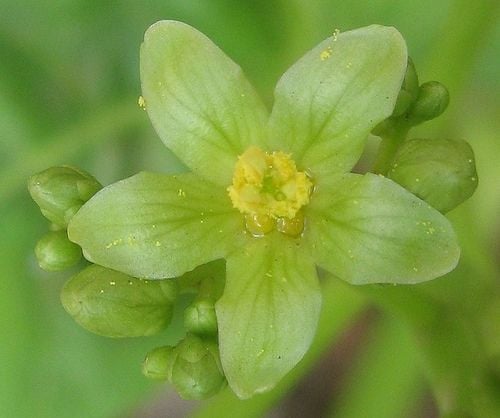This close-up photograph captures a beautifully centered green-petaled flower in full bloom, prominently displaying its intricate details. The flower features five light green petals radiating from a vibrant yellow center, which is dusted with pollen, indicating recent visits from pollinating insects. Delicate veins are visible on the petals, adding texture and depth to the image. Surrounding this main flower, there are numerous green buds in varying stages of readiness, suggesting an impending bloom of similar flowers. The background is artfully blurred, with hints of green leaves and stems, enhancing the focus on the flower. Subtle red sections at the bottom of the picture add a touch of color contrast, although they remain out of focus, blending harmoniously with the overall green backdrop.